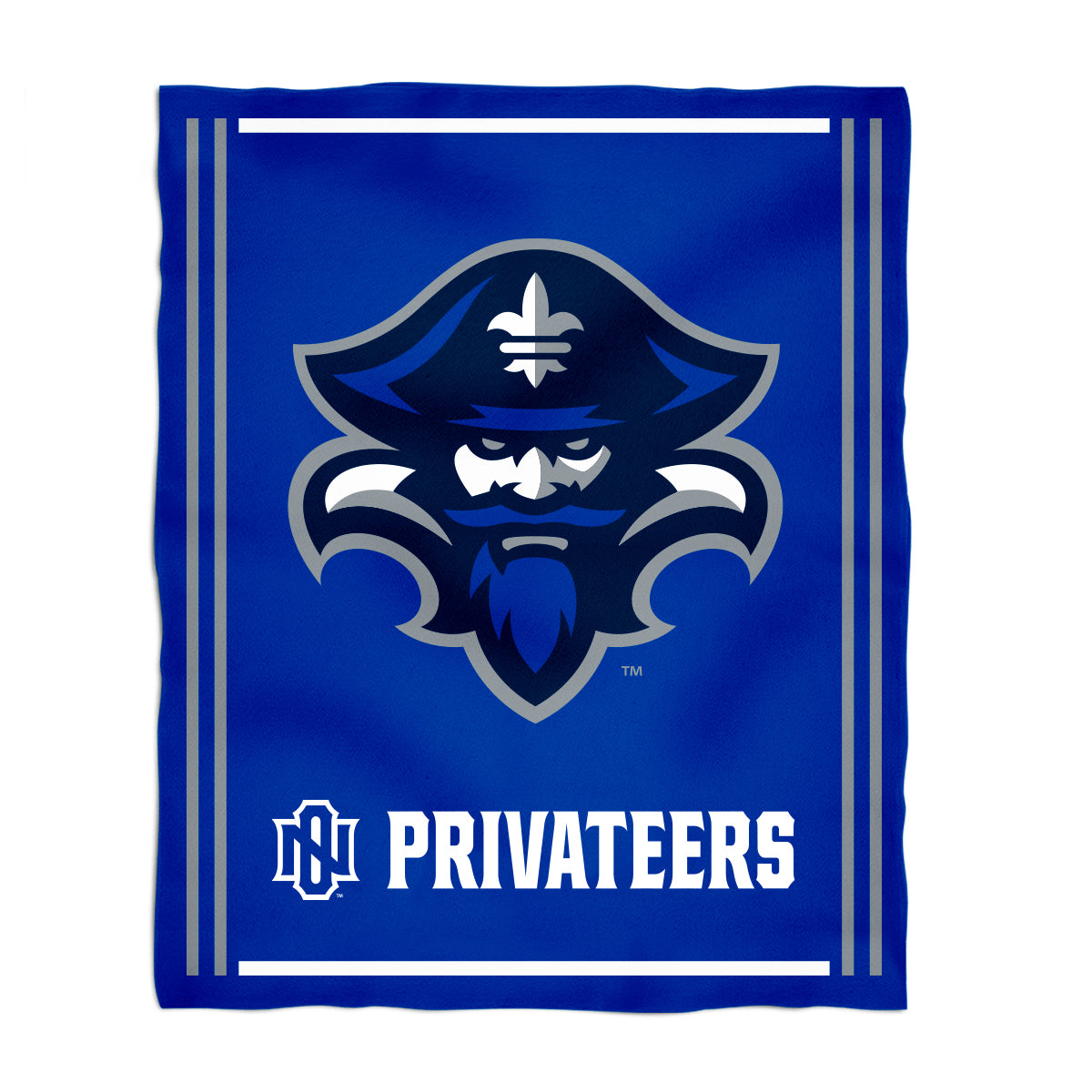This image is a graphic resembling a sign or flag, predominantly featuring dark to medium blue hues with a textured appearance and uneven borders. It has a distinctive layout with two thin, vertical gray stripes running nearly the full height on the left and right sides, complemented by thin white horizontal borders at the top and bottom edges.

The central focus of the graphic is a stylized depiction of a pirate-like figure. This character sports a blue beard and mustache, and wears a traditional pirate hat reminiscent of Napoleon’s, adorned with a white and gray emblem resembling a fleur-de-lis. The pirate’s stern gaze is directed at the viewer. 

Beneath this character, in bold white capital letters, the word "PRIVATEERS" is prominently displayed. To the left of the text, the abbreviation "N-O", possibly indicating New Orleans, is featured, underscoring the graphic's likely connection to a school or team whose mascot is the Privateers.